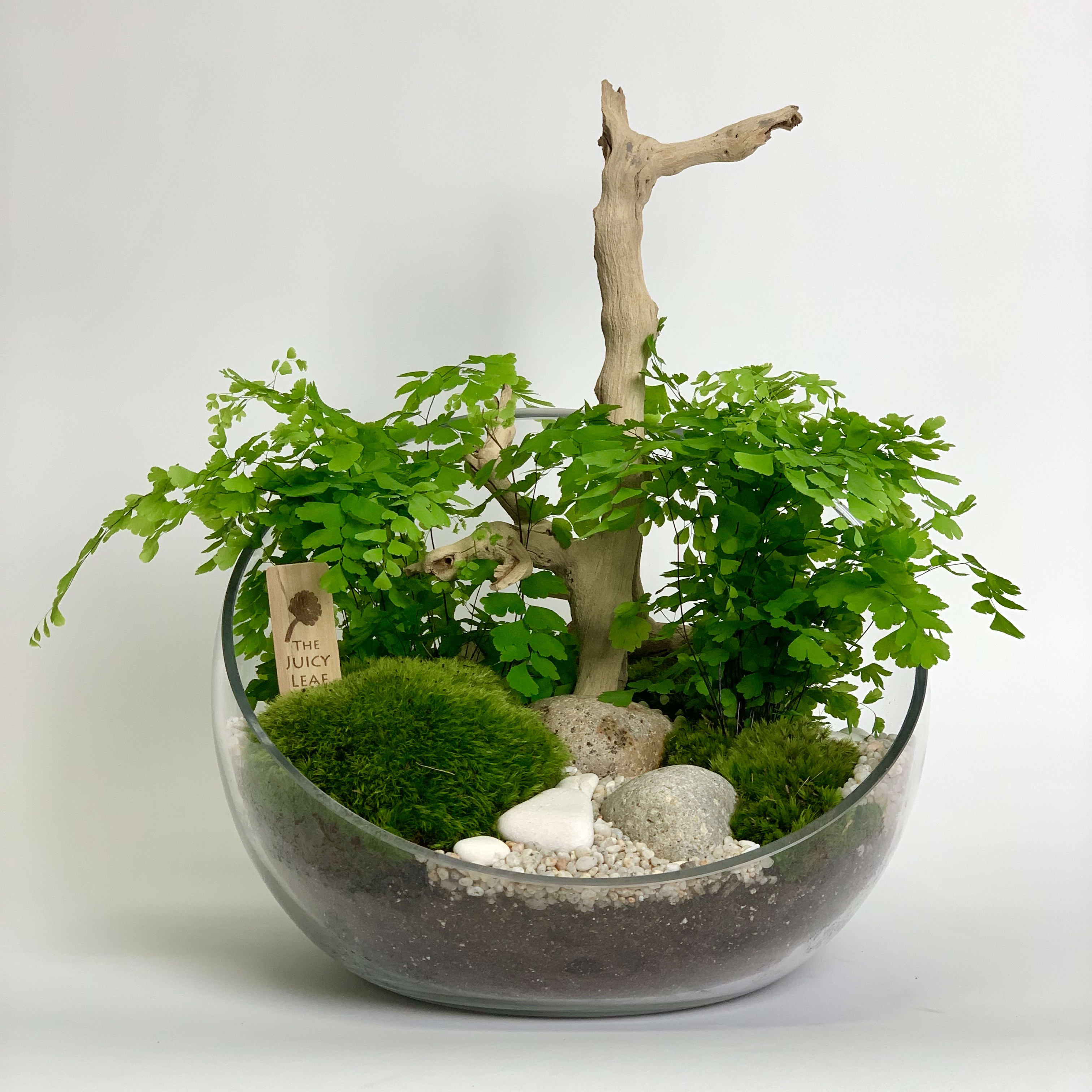The image showcases a unique potted plant arrangement within a clear glass semi-circular bowl, with the front cut at a lower angle than the back. The base of the pot contains a layer of dark brown soil topped with small white rocks, and above that, larger white rocks, two on the left and one grayish rock on the right. Rising from the center is an artificial tree branch adorned with small plant leaves. To the left of the branch, there's a lush green patch with grass and larger fern-like leaves, while the right side features plants of a darker green-brown hue. Nestled among the greenery is a light wooden sign with a face illustration and the text "The Juicy Leaf." The setup sits on a white surface with a white background, and a light source from the right casts a shadow to the left, accentuating the glass bowl's transparency and the intricate details of the plant display.